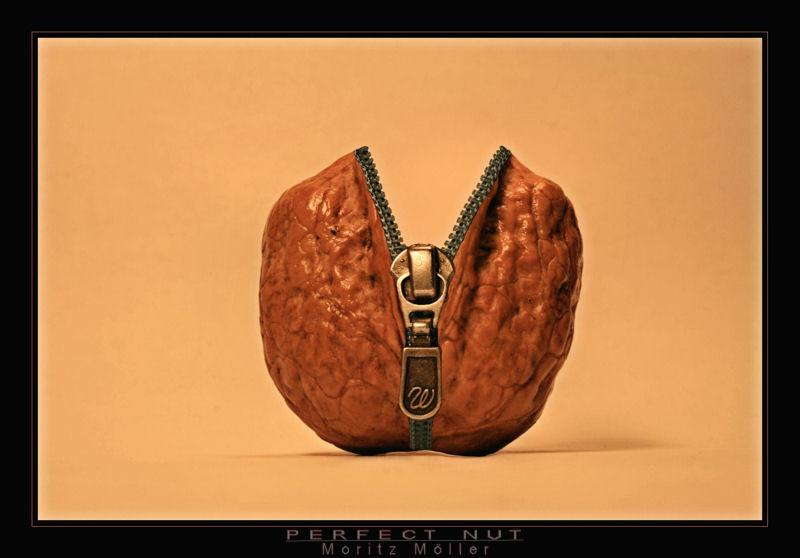The image is a modern artwork centered around a detailed walnut, set against a solid, sandy orange background with a slight drop shadow at its base. This walnut, light brown with darker undertones, stands out as the primary focus and is meticulously depicted with a realistic, shiny texture. The walnut is uniquely split in half by a brass-colored metal zipper, which is halfway unzipped, revealing an intriguing interior. The zipper handle, adorned with a cursive "W," adds a distinctive touch to the composition. Below the artwork, the caption "Perfect Nut" is presented in a light white-blue font, accompanied by the artist's name, "Moritz Mahler," emphasizing the piece’s playful yet intricate design. The image is framed with a black border, suggesting it is part of a gallery or art show exhibit.